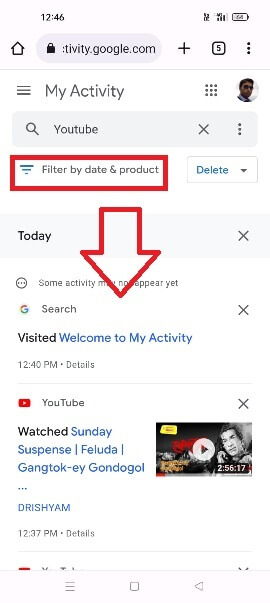The image shows a detailed screenshot of the "My Activity" page on activity.google.com at 12:46 PM. Central to the image is a series of UI elements beginning with the depiction of a house icon adjacent to a gray search bar area. The search bar contains the URL activity.google.com, with a plus sign next to it, followed by an icon of a square featuring the number five.

Below this header, the page displays the title "My Activity," alongside another search bar pre-filled with the term "YouTube." Highlighted in red is a second search bar, also featuring the term "YouTube." Beneath these, options to filter by date and product are available, indicated by a downward-pointing arrow. This arrow leads to a section indicating a visit at 12:40 PM, labeled "Welcome to My Activity," with a "Details" option next to the time stamp.

The image further includes the recognizable YouTube logo—a red rectangle with a white play arrow. Adjacent to this logo, or just below it, are the words "Watched Sunday Suspense," with the timestamp of 12:37 PM. The associated video has a duration of 2 hours, 56 minutes, and 17 seconds.